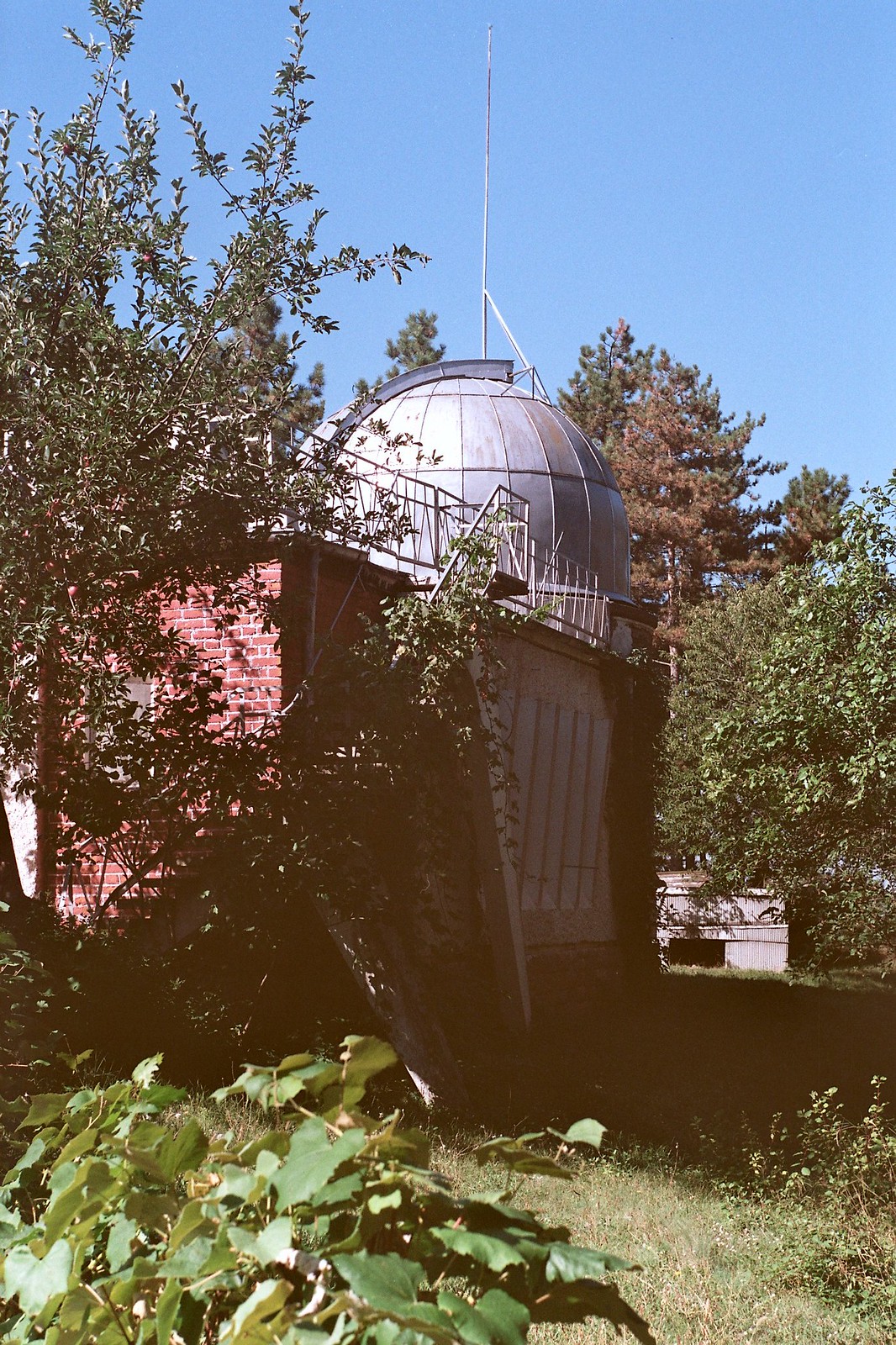The image captures what appears to be an older, small observatory tower set within a lush, wooded area. The structure features red brick walls at its base, indicative of its connection to a larger building. A silver, semi-spherical dome sits atop the brick foundation, crowned with a slender metal pole or antenna protruding from its center. The tower also has a small railing suggesting the presence of a stairway or entrance leading to the dome. In terms of setting, the observatory is surrounded by diverse flora, including grass, small bushes, and an array of trees displaying shades of green and brown. The sky is a clear, vivid blue, enhancing the overall clarity of this serene, nature-filled scene. The photo evokes a sense of nostalgia, hinting at its age through both the structure and the natural landscape that envelops it.